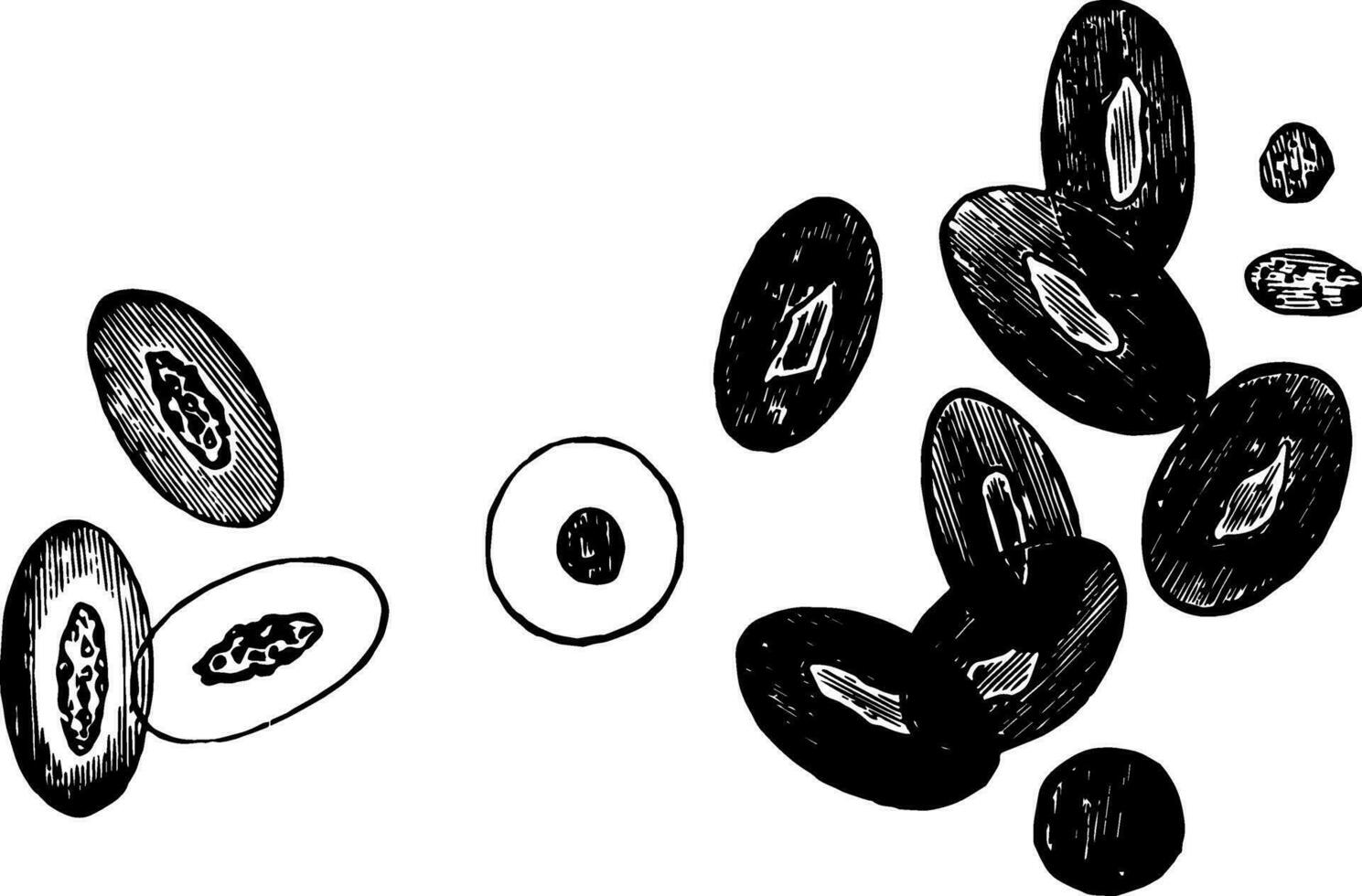This detailed black and white sketch depicts an assortment of 14 various oval and circular shapes, potentially resembling albums or discs, beans, buttons, or even blood cells. The ovals on the right are mostly black with a white center, crisscrossed by black lines. One of the ovals appears to be a child's face sticking its tongue out with a possible dog figure beneath it, featuring an eye, mouth, and nose with horizontal lines. To the left, there are seven oval shapes resembling LPs, characterized by a black outer ring and an inner white circle with black lines. Below these is a smaller, perfect black circle. Directly left of this black circle is another oval with black and white concentric circles. One oval nearby is predominantly white with black dots and heavy lines. Higher up at an angle, overlapping ovals showcase various shades of gray with distinctive line patterns. The entire composition is intricate, combining elements that are detailed with pen and ink, offering a complex and abstract interpretation.